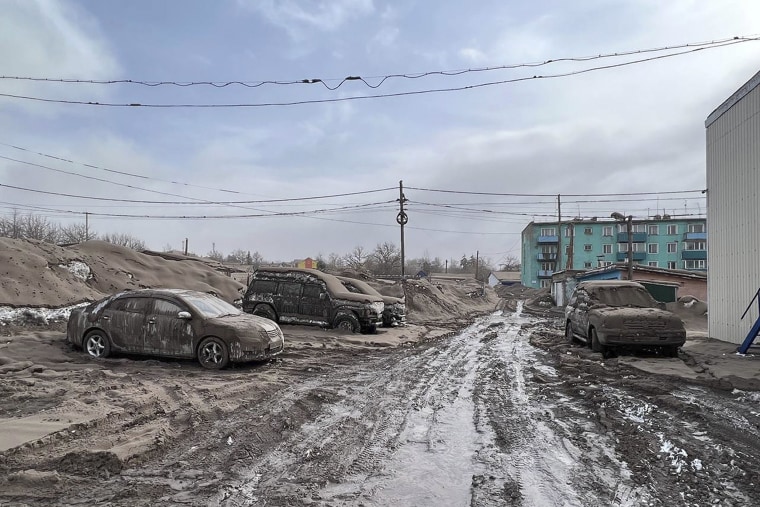The image depicts a muddy outdoor environment, likely the aftermath of a flood or natural disaster. In the center, there is a waterlogged, muddy road flanked by cars covered in thick layers of mud. On the left side of the road, three mud-caked cars are parked in a line facing right, with barely any of their surfaces visible due to the extensive mud. On the right side of the road, a single car, similarly encrusted with mud, faces the viewer. The right side of the image also features two buildings: a white or grey structure closest to the camera with a blue staircase, and a larger, teal-colored, multi-storied building with several windows farther back. The backdrop includes various trees and a cloudy sky. Overhead, power lines stretch across the scene, adding to the sense of a disrupted, disaster-stricken landscape.